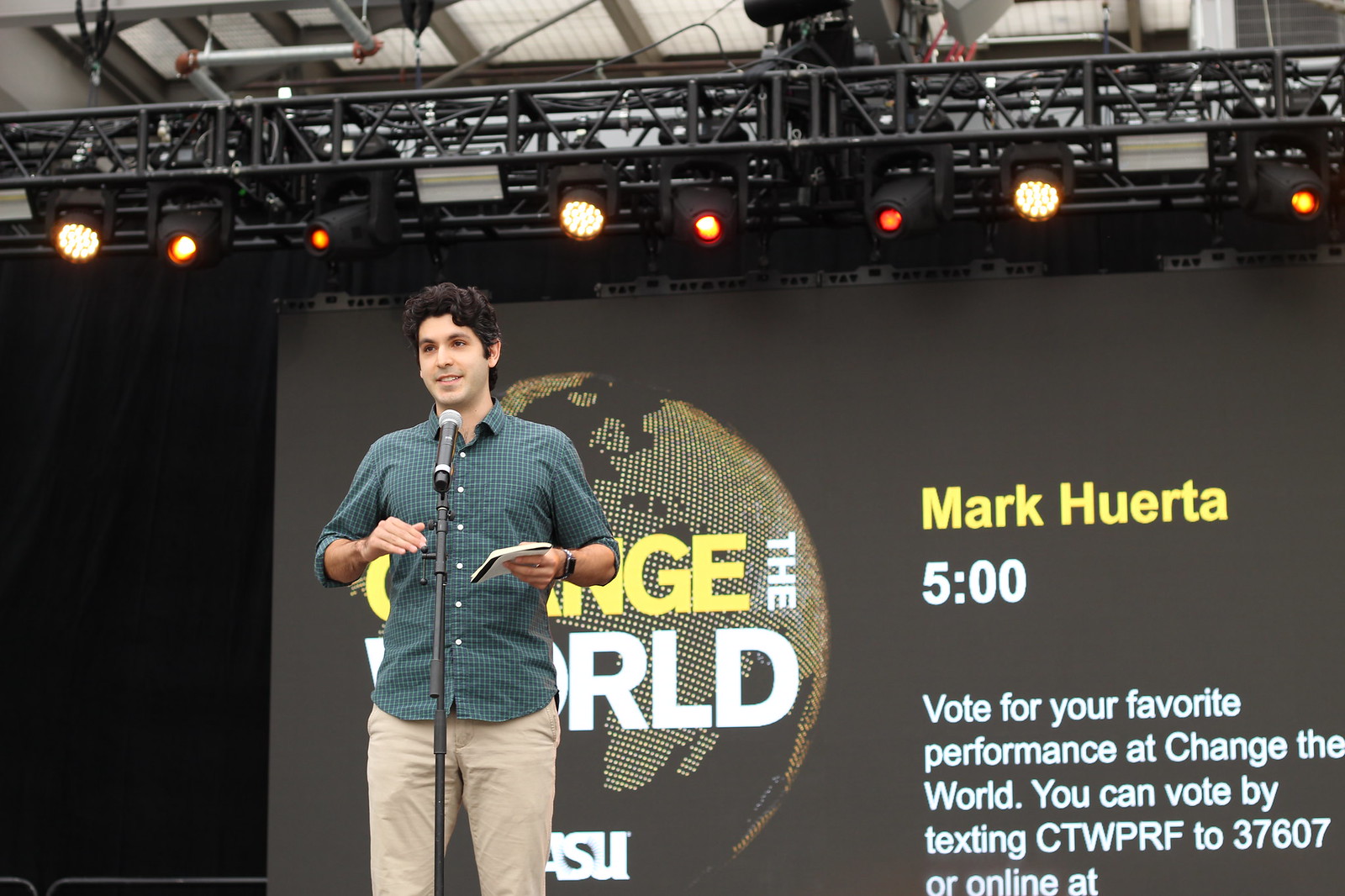The image depicts a man on a large stage, surrounded by black scaffolding adorned with multiple forward-facing spotlights. Above the stage, a white roof is visible, with glimpses of a gray ceiling or sky peeking through the scaffolding. The backdrop is a prominent LED screen divided into two sections: the left side features the words "Change the World" with a stylized pixelated globe behind them, while the right side displays "Mark Huerta" in yellow font and "5pm" in white font. Beneath this text, there is an invitation to vote for the favorite performance by texting "CTWPRF" to 37607 or online. The man on the stage is wearing a green plaid shirt and beige pants, and he is speaking into a microphone.